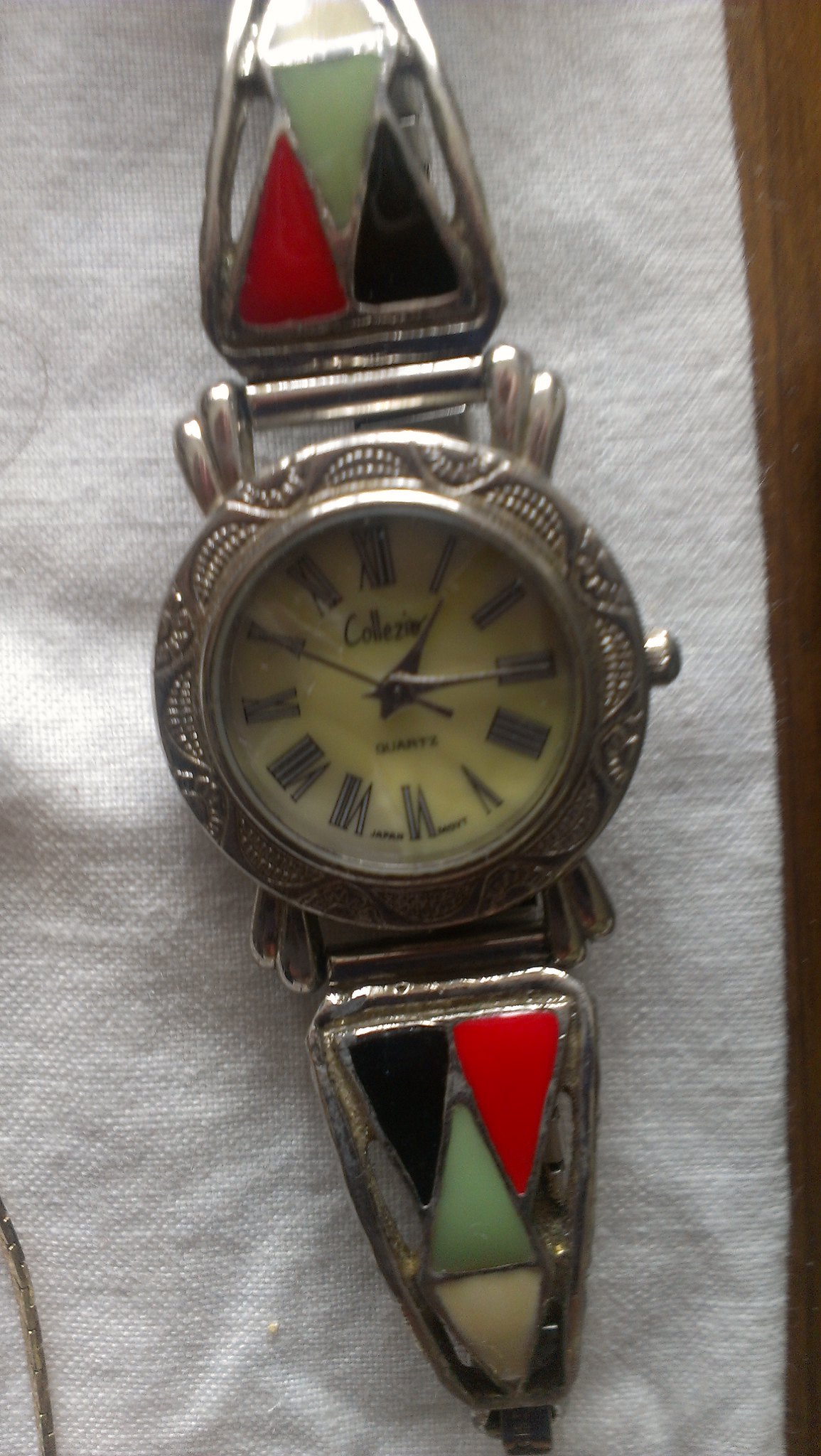This image features an antique-styled pocket watch, which might also function as a pin. The watch rests on a piece of white cloth draped over a table. The watch's casing appears to be made of pewter, characterized by a triangular form at both the top and bottom.

Contained within these silver pewter triangles are three smaller triangles in distinct colors: red, white, and black. Additionally, there is another triangular design at the end, comprised of red, green, and black sections, complemented by white accents at the edges.

Surrounding the watch face is an intricately detailed etching with a wavy pattern, adding an element of elegance to the piece. The watch face itself has a beige background and features Roman numerals to indicate the time. It bears the inscription "Quartz," and beneath this, the word "Japan" can be seen, suggesting its place of manufacture.

The brand name on the watch is partially legible, appearing to spell "COLLEZI," with the last few letters somewhat ambiguous, possibly forming "ER" at the end.